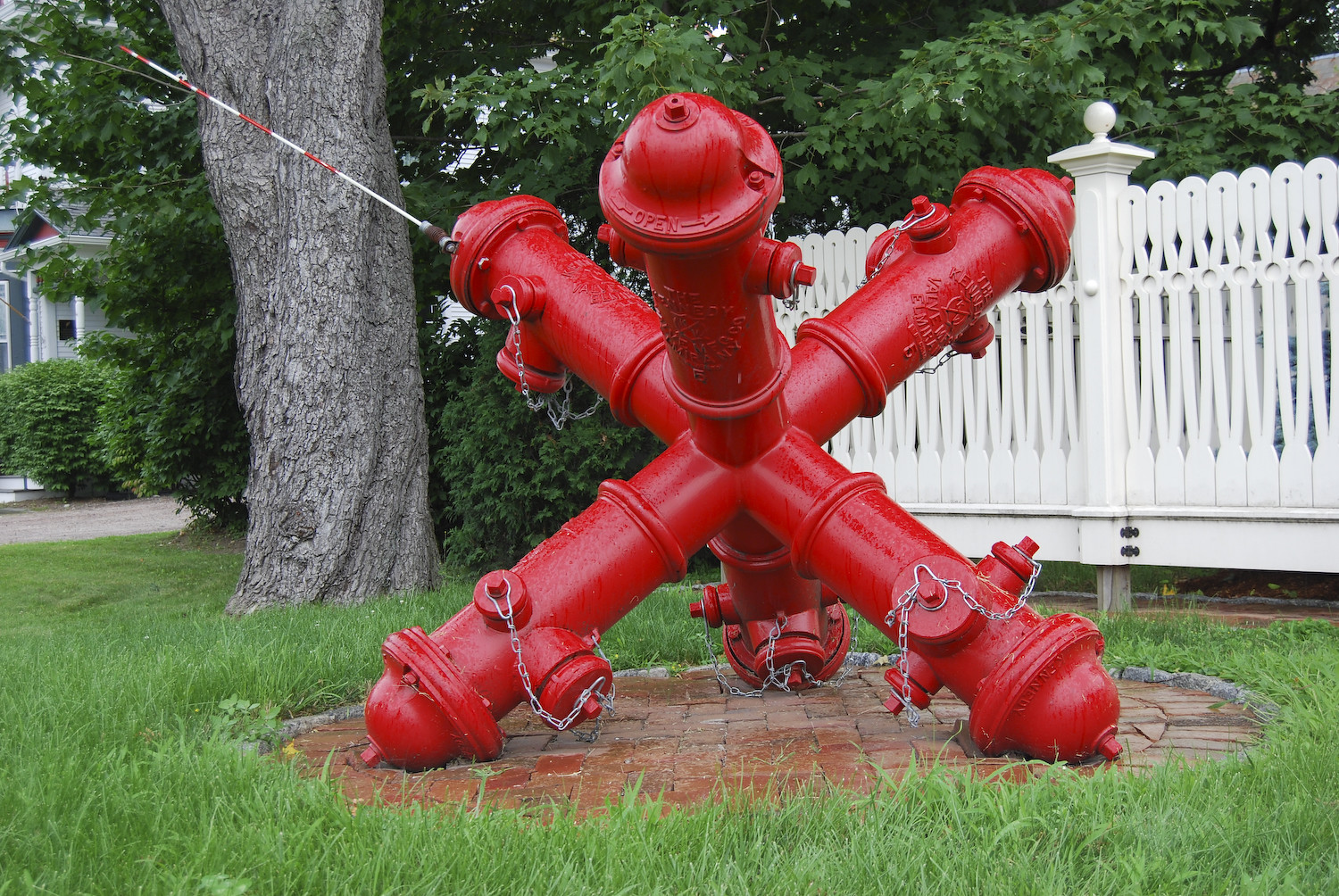The image depicts a vibrant red fire hydrant sculpture designed to resemble the classic children's game jacks. The sculpture consists of multiple fire hydrants interconnected at their bases, forming an X shape with hydrants extending from each side, mimicking the appearance of jacks. All the hydrants feature silver link chains attached to their side knobs. One of the hydrants has a red and white tether, possibly for support. This unique art piece is situated atop a circular red brick platform, surrounded by lush green grass. In the background, there is a wooden white picket fence, and lush greenery, including shrubs and trees. A portion of a house is visible to the left, partially obscured by a large tree.